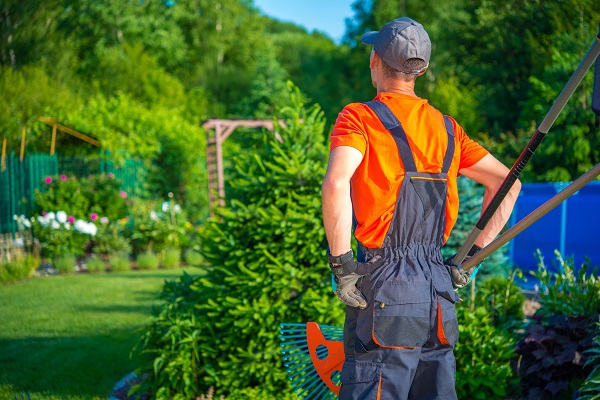The image captures a sunny outdoor scene featuring a man who appears to be a gardener, standing in the right foreground of the photograph. The man is dressed in blue polyester-style overalls with a cinched waist and multiple cargo pockets, the inner parts of which are lined with orange fabric. He also wears an orange short-sleeve shirt and a gray baseball cap. Thick gray and black gardening gloves rest on his hips, and in his right hand, he holds the wooden handle of a green and orange rake along with a black and silver handle of another gardening tool. The man, facing away from the camera, directs his gaze towards the garden.

The background, slightly out of focus, displays a rich green landscape with trees and a trellis standing prominently in the center. Various plants are visible, including bushy green foliage, white and pink flowers, and a well-mowed green lawn. Towards the right side of the frame, a faint outline of what appears to be an outdoor pool can be seen alongside some blue containers in the distance. The lower left portion of the image reveals grass and more flowers, adding to the serene and meticulously maintained garden setting.